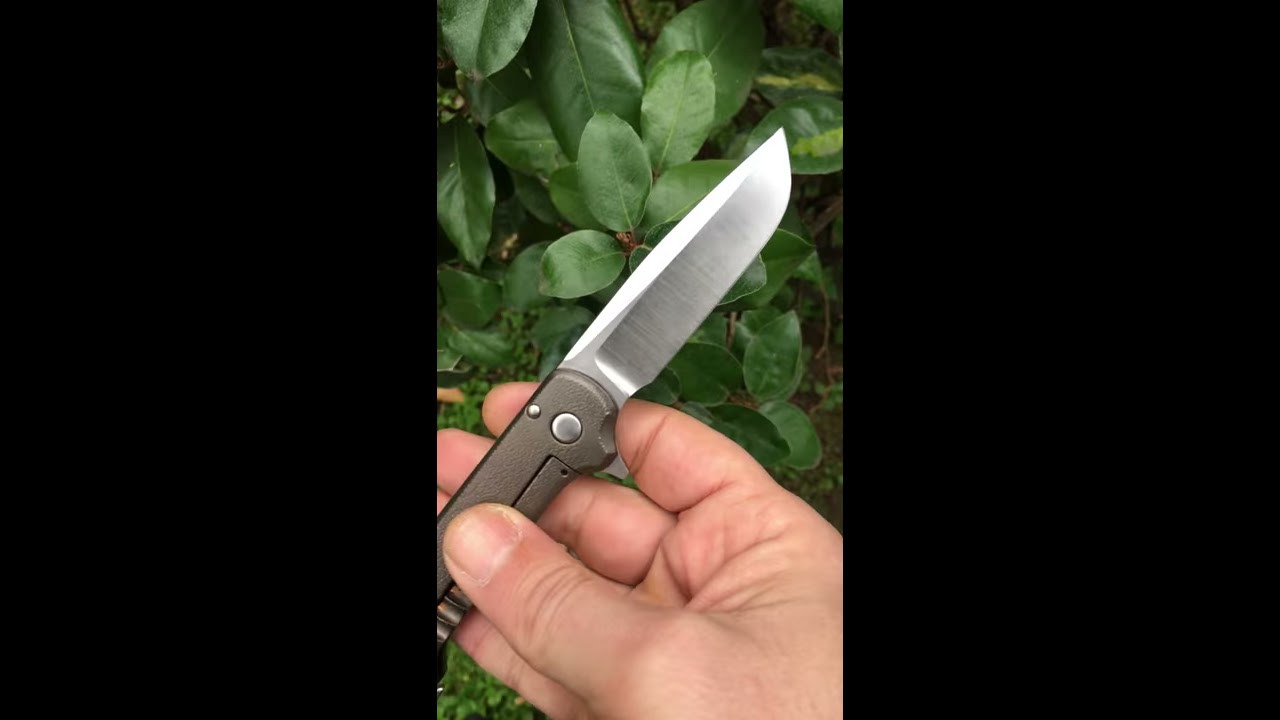This detailed close-up photograph captures a light-skinned individual's hand, likely belonging to a white or Asian man, clutching a small pocket knife with a black handle and a brushed, stainless steel blade that measures approximately two to four inches in length. His thumb is positioned over the base of the knife, suggesting a secure grip despite the compact size of the handle, which only accommodates a few fingers. The backdrop consists of lush, dark green leaves, indicating an outdoor setting with natural sunlight filtering through. Additionally, the image features black rectangular framing on both sides, contributing to a focused, narrow composition. There is no text in the image, directing full attention to the knife and the hand that holds it.